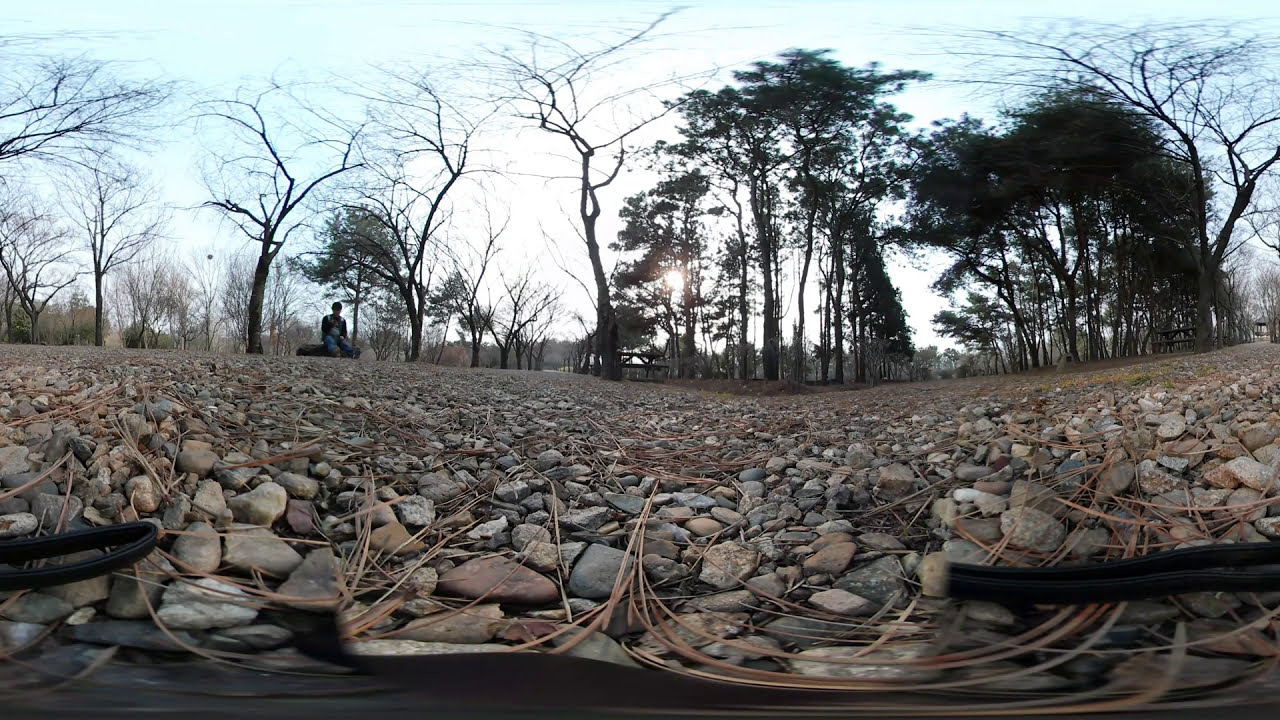In this image, a rocky field extends across the entire bottom half, with stones and pebbles interspersed with dead pine needles. The rocks vary in color from gray to light brown to dark brown, gradually blending into the earthen colors near a cluster of trees in the middle distance. The trees are a mix of tall, skinny ones with some leaves and dead trees with bare branches, indicating a fall setting. Toward the left side of the image, a person in blue jeans sits on a brown object, possibly a bench or a log, gazing out over the landscape. The sky is light blue with white clouds, occupying the top portion of the image and enhancing the open, daytime outdoor atmosphere. The horizon line, slightly curved in the middle, separates the rocky foreground from the trees and sky background.